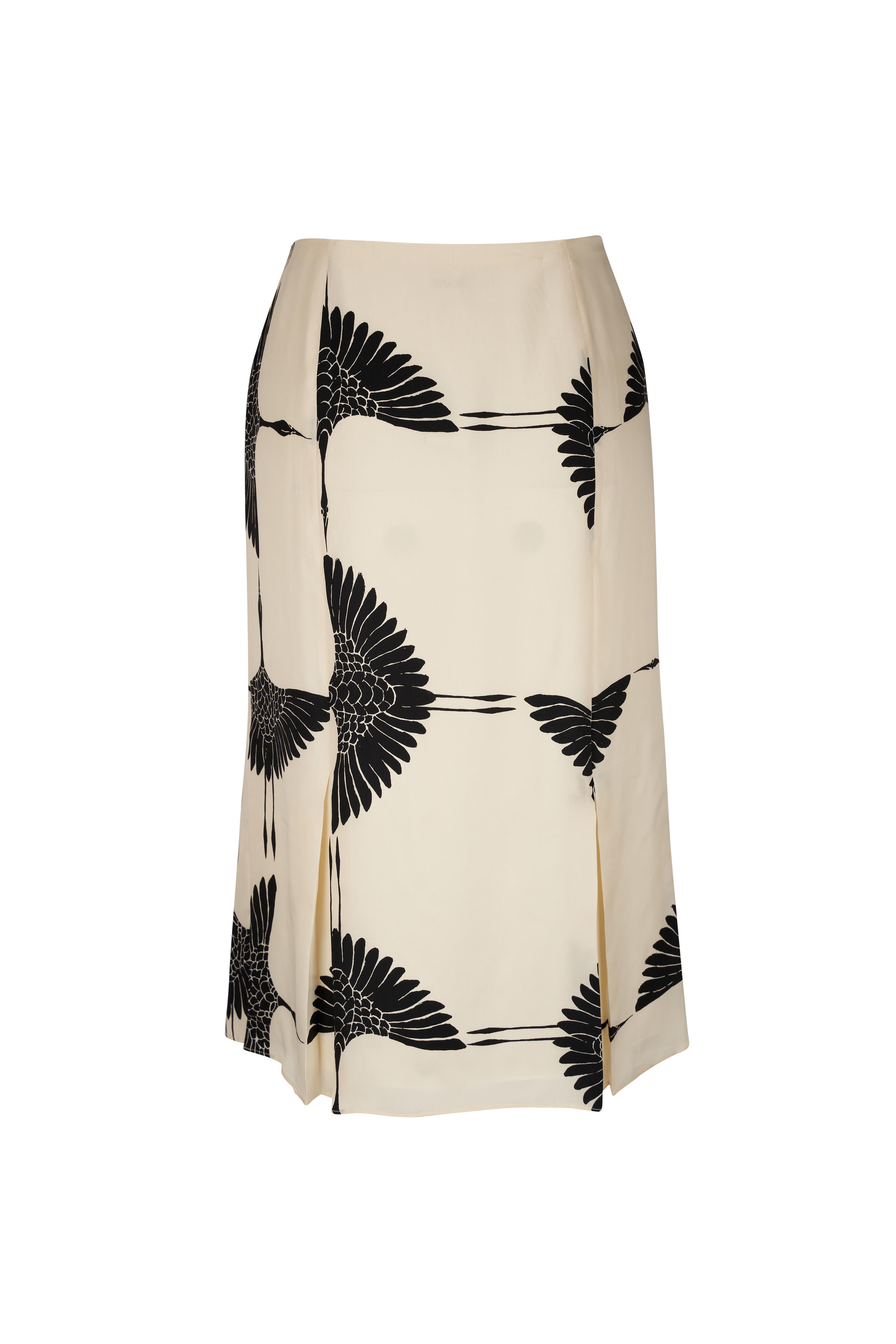This photograph showcases a cream-colored skirt displayed against a stark white background. The skirt, appearing to be made from a thick, rigid linen material, features prominent pleats—one on the left and another on the right. Adorning the skirt is a repetitive decorative pattern of black birds, possibly stylized cranes, characterized by their elongated thin legs and fanned-out feathers. The bird motifs stretch across the front panel and over the pleats, creating an engaging visual continuity despite some cut-offs in the design. The black bird drawings, simplistic rather than realistic, stand out distinctly against the cream fabric, forming a striking contrast. The image focuses solely on the skirt, with no text or additional elements present.